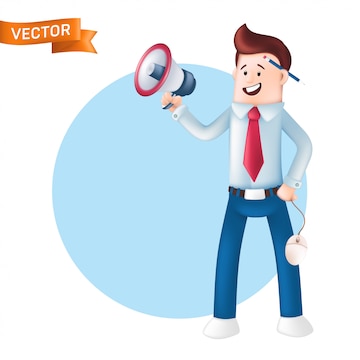This image is a cartoon-style drawing set against a white background with a small orange banner in the top left corner, displaying the word "VECTOR" in white capital letters. The focal point is a stylized, joyful man standing in a light brown circle. He is depicted with long, straight legs clad in blue pants and white shoes. He sports a white button-down shirt paired with a red tie that hangs just above his silver-buckled belt. His face, which emerges directly from the collar without a visible neck, features two eyes, raised eyebrows, a corny grin with front teeth showing, and a mouth slightly off to the right. Atop his head is a swirl of brown hair, and a blue pencil is tucked behind his left ear. His left hand is held to his hip, supporting a cord that ends in a computer mouse dangling just above his knee. His right arm is extended outward, holding a megaphone that is white with a blue mouthpiece and a red ring around the end. The man appears to be speaking or shouting into the megaphone with a sense of enthusiasm.